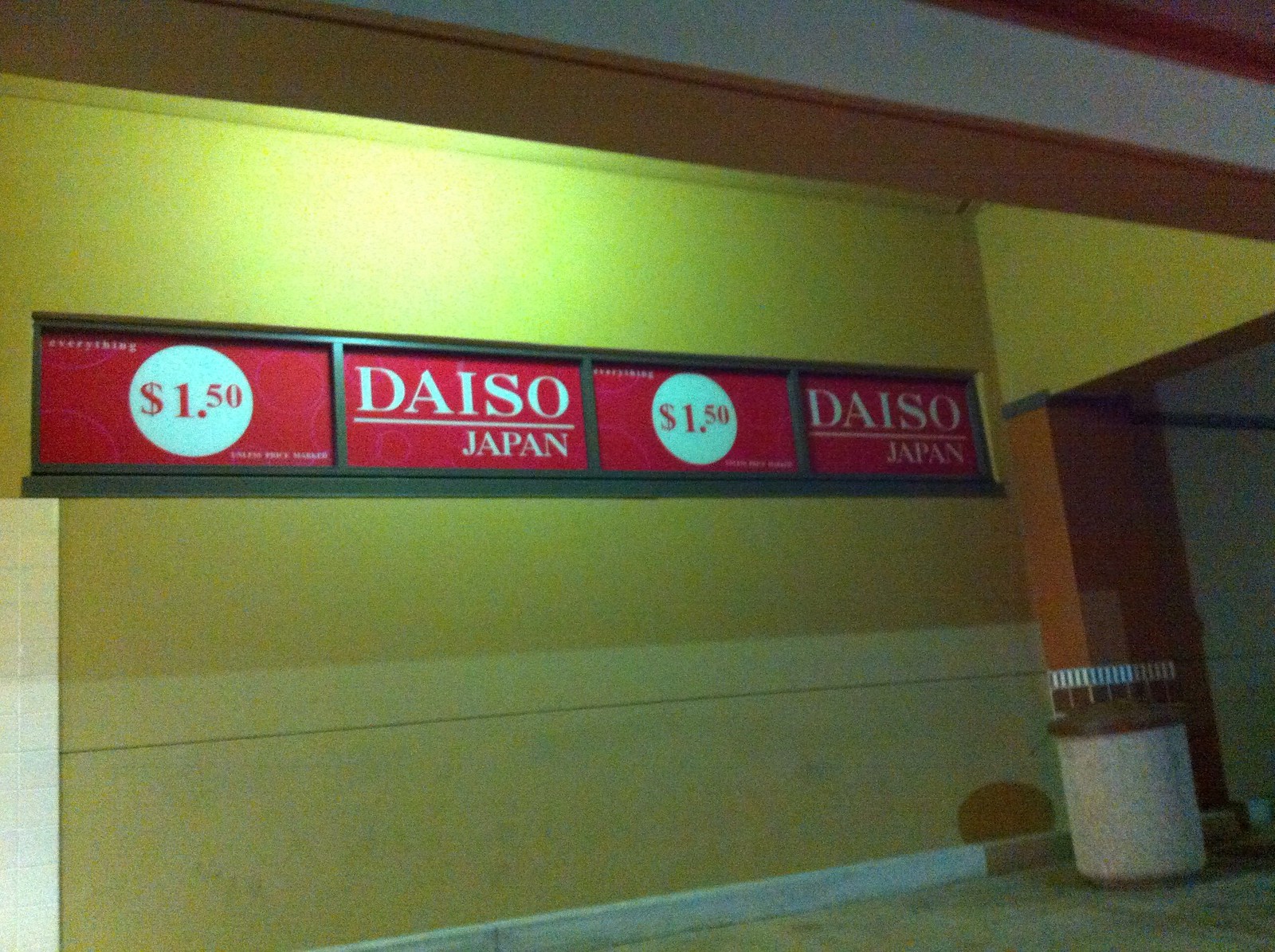The image depicts the exterior of a Daiso Japan store, situated in an alleyway or possibly a parking garage area. The prominent feature is a large sign with a yellow background and bold red text indicating "Daiso Japan." Central to the sign is a white circle displaying "$1.50," highlighting the store's pricing policy. The sign combines red and white elements effectively to convey the message. Surrounding the building, there are concrete columns and a ceiling, indicative of a parking structure. The ground appears dirty and is marked with white linings. Scattered around, there are multiple trash cans, including a large outside stone trash bin. The area is illuminated slightly at the top, with a mix of white and brown hues visible on the walls and floors, further underscoring the gritty atmosphere of the location.